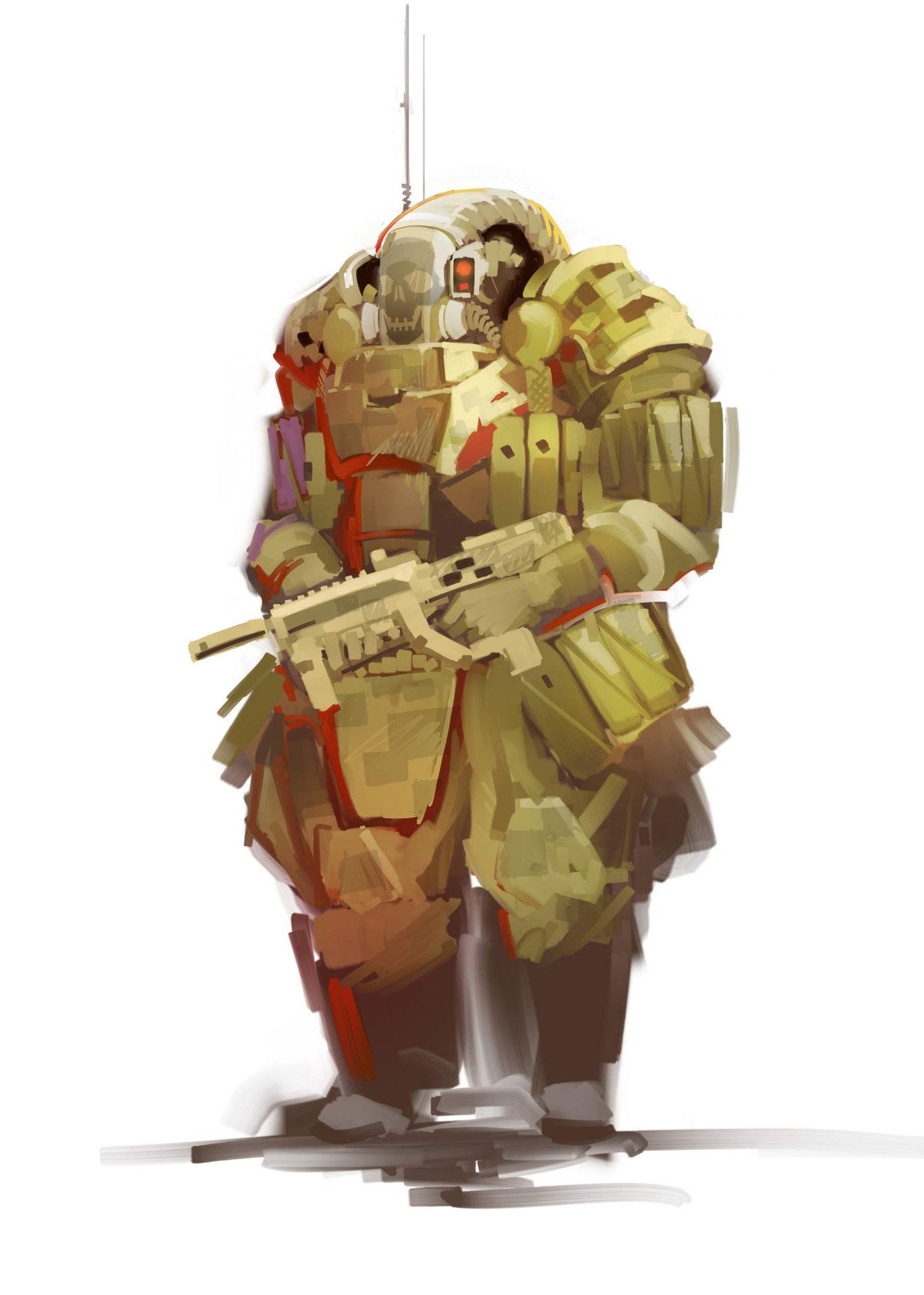This is an illustration of a futuristic, heavily-armored character, likely from a concept for a movie or video game. The character is depicted standing in a white background, wearing a bulky, tan and gold military suit, segmented for added protection and flexibility. The armor is adorned with red accents, and features black boots. The helmet of the suit is adorned with a gray human skull design on its front and is equipped with an array of gadgets, including two antennae, tubes, and lights. The eyes of the helmet are stylized as orange circular lights. The armored figure is holding a blocky, tan-colored assault rifle with a wide trigger area, cradling it with both hands, facing slightly to the left. The overall art style is digital, with broad, solid brush strokes giving it a sketchy yet detailed appearance. The character looks menacing and ready for battle, embodying a sci-fi aesthetic.